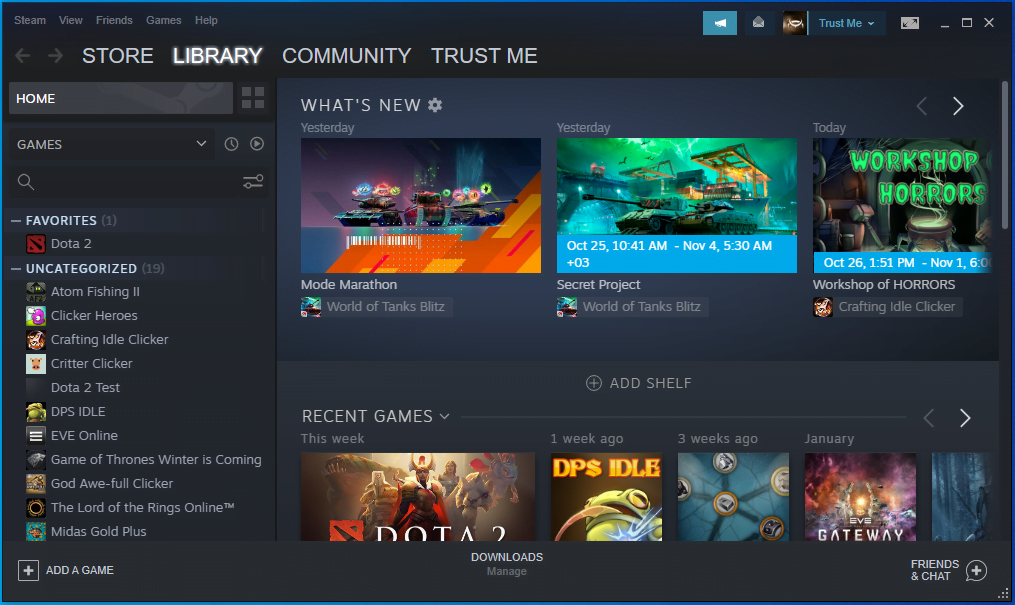A detailed screenshot of a Steam library interface is displayed, featuring the platform's characteristic shale gray background. In the top left corner, the familiar Steam menu options are visible: "View," "Friends," "Games," and "Help." Just beneath these, the main navigation tabs are prominently shown in capital letters: "Store," "Library," "Community," and "Profile," with "Library" currently selected.

Directly below the primary navigation, there's a bar listing "Home" and "Games." The "Home" section is highlighted, followed by the "Games" section which includes two categories: "Favorites" (displaying one game, Dota 2) and "Uncategorized" (host to nineteen different games). The games visible in the "Uncategorized" list are "Adam Fishing," "Clicker Heroes," "Crafting Idle Clicker," "Critter Clicker," "Dota 2 Test," "DPS Idle," "Eve Online," "Game of Thrones: Winter is Coming," "Godawful Clicker," "The Lord of the Rings Online," and "Might & Magic: Heroes VII."

In the bottom left-hand corner of the interface, there's a button labeled "Add a game," providing users the option to expand their library further.

On the right-hand side of the screen is a widget labeled "What's New," accompanied by a gear icon for settings. This section highlights various game updates and headlines. Currently featured are:

1. A visual showcasing "Mode Marathons" with a dynamic image of two tanks, surrounded by bright, revolving objects.
2. "Secret Project: World of Tanks Blitz," displayed with an image of a tank set against a futuristic backdrop.
3. "Workshop Core," presenting an image that looks like an old-fashioned workshop filled with tools and machinery.

This detailed visual representation of a Steam library provides insight into the user's collection and recent updates in the gaming world.